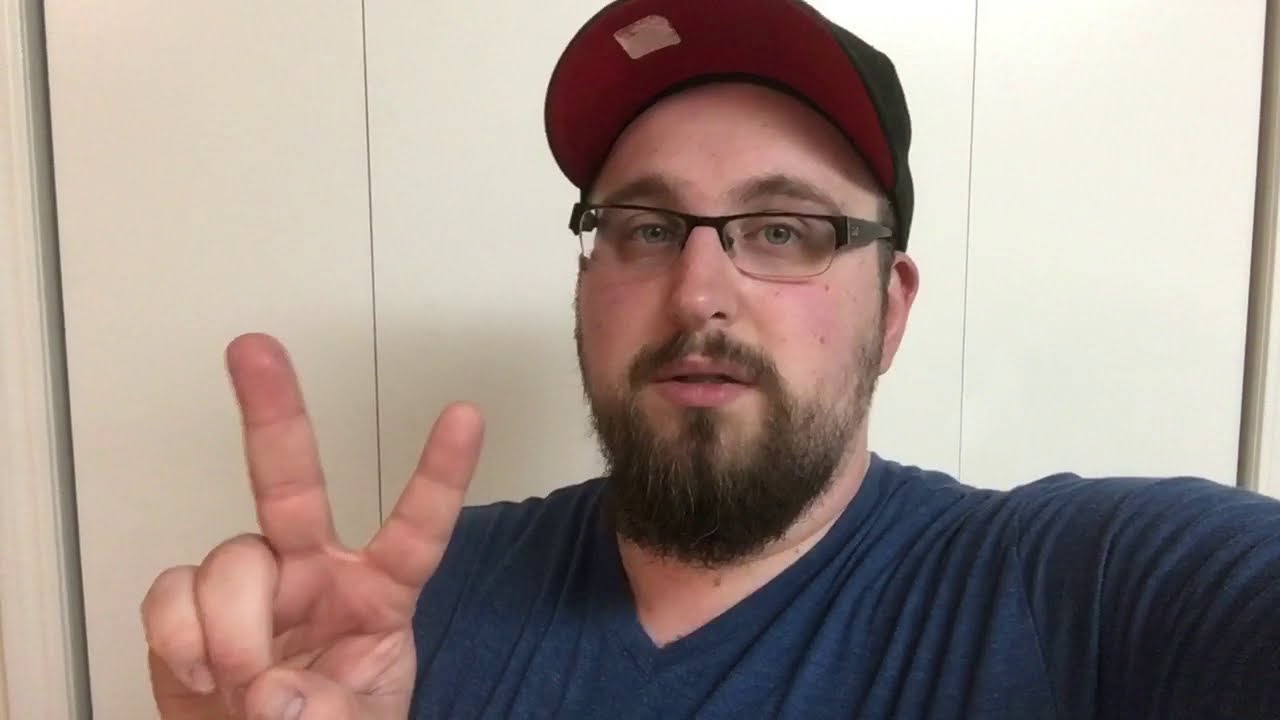The image captures a Caucasian man taking a selfie, his left arm extended and mostly out of view. He's making a peace sign with his right hand, revealing his thick, wide fingers and chewed-up nails. The man has slightly pale skin, blue eyes, and wears half-rimmed black glasses. His brown hair is mostly hidden under a black hat with a red under-rim and an old price sticker attached. His dark brown beard has a few strands of gray, and he sports bushy, messy brown eyebrows. He’s dressed in a loose-fitting navy blue V-neck cotton t-shirt. The background features a closed white folding closet door and an adjacent white wall with visible panel lines.